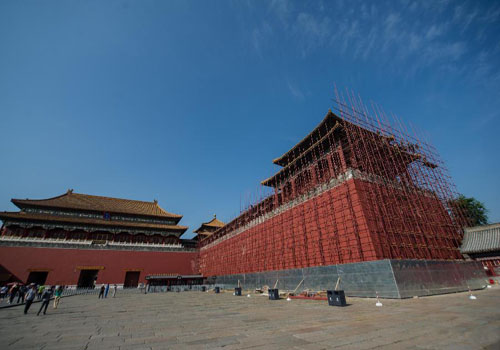The image depicts an outdoor scene, possibly in an Asian country, featuring a distinctive architectural style characterized by pointy roofs. The roofs are sharply angled, converging to pointed ends. The photograph appears to be taken from ground level, providing a clear view of the structures above. The buildings are predominantly red, with a white streak running horizontally around them. Several people are present, seemingly tourists, as they gaze at the impressive architecture. The ground to the left is cement gray, suggesting a well-trodden path or plaza. On the right side, there are signs of ongoing construction, including bolts, fences, and bins for holding materials, but no workers are visible. The scene captures a moment of stillness amidst the blend of historical and modern elements.